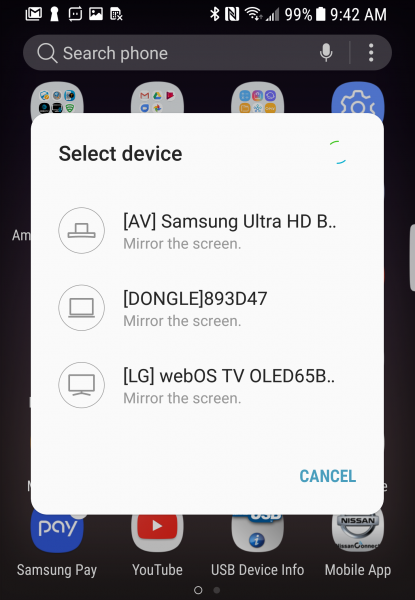This image showcases a screenshot of a smartphone with multiple apps running simultaneously. At the very top of the screen, familiar app icons are displayed, indicating the presence of Google services like Gmail from left to right, followed by icons representing messaging, photos, an unspecified application, Bluetooth connectivity, Wi-Fi status, and network signal strength. The battery is nearly full at 99%, and the time is 9:42 AM.

Directly below the top icons, the search functionality is visible, which includes a password search option, a microphone for voice search, and a general phone search bar. The home screen contains around 20 different app icons, although only four are distinctly identified near the bottom of the screen. These visible apps, arranged from left to right, are Samsung Pay, YouTube, USB Device Info, and Mobile App.

Dominating the screen is a message prompt titled "Select Device" with three available options for connection. The first option reads "AV Samsung Ultra HD, B..." hinting at an incomplete text. The second option is labeled "dongle, D-O-N-G-L-E-8-9-3-D-4-7," and the third option states "LG Web OS TV O-L-E-D-6-5-B." Additionally, there is a cancel option at the bottom of the select device prompt, allowing the user to exit the selection process.